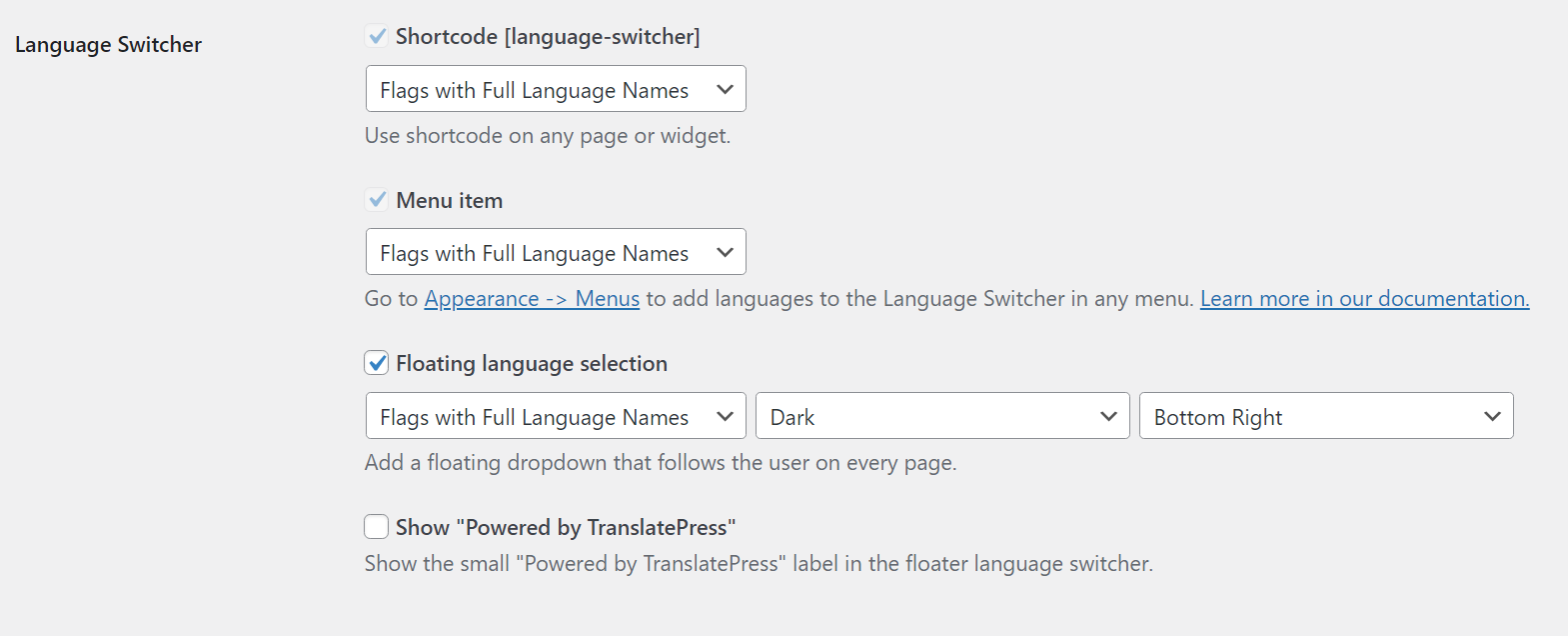In this image, the background is a grayish color, providing a neutral backdrop for the content. At the top left of the image, the words "Language Switcher" are prominently displayed, followed by an empty space below. To the right of "Language Switcher," there is a small square box with a check mark accompanied by the word "Shortcode," and in brackets next to it, the words "Language Switcher" appear again.

Below this section, there is a text box that reads "Flags with Full Language Names." Underneath, there is a sentence stating, "Use shortcode on any page or widget." Moving further down, another checkbox is marked with a checkmark and labeled "Menu Item." Directly below, there is another text box with the same phrase, "Flags with Full Language Names."

Following this, the instructions "Go to Appearance" are visible, highlighted by an arrow pointing to the word "Menus," which is also highlighted in blue. The text continues, "To add languages to the language switcher in any menu, learn more in our documentation," with both "learn more in our documentation" and "Appearance to Menus" colored in blue to signify clickable links.

Further down the image, there is another square with a checkmark labeled "Floating Language Selection" along with three options arranged in boxes. The first box again states "Flags with Full Language Names," the second box is labeled "Dark," and the third one reads "Bottom Right." 

At the very bottom of the image, there is an unchecked box labeled "Show Powered by Translate Press."